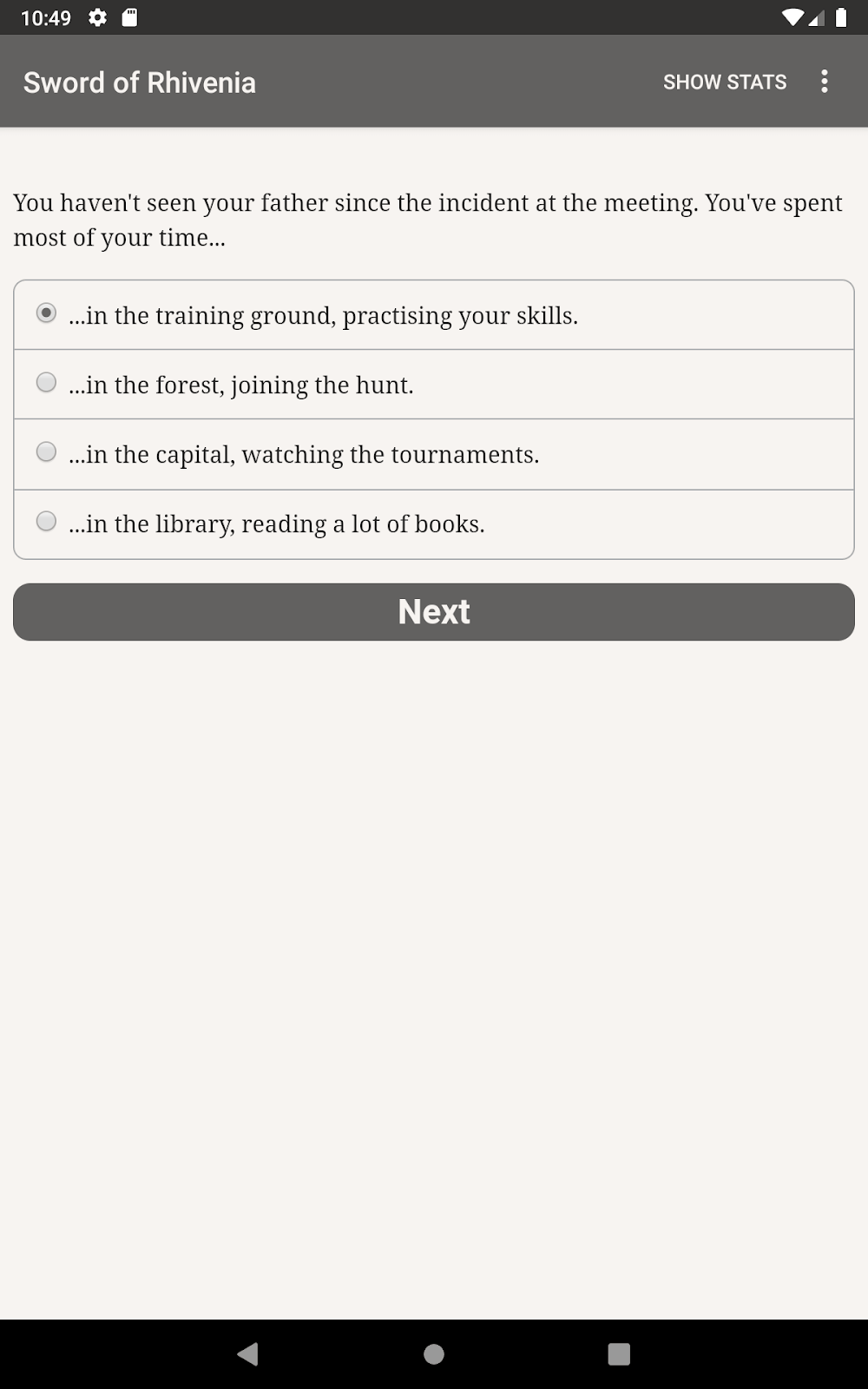The image is a screenshot captured from the display of a mobile device, likely a cell phone or an iPad. The device's status bar at the top indicates it is 10:49 AM, shows various settings and icons, and confirms a full battery charge. 

Dominating the top portion of the screen, a gray header contains the title "Sword of Ravenia" on the left, while towards the right, it says "Show Stats" followed by three vertical white dots. Beneath this header, within a tan textbox, there is an ongoing narrative: "You haven't seen your father since the incident at the meeting. You've spent most of your time..."

Below this text, there are multiple interactive choices for the user to select from:
1. "...in the training grounds, practicing your skills." (Which is already selected)
2. "...in the forest, joining the hunt."
3. "...in the capital, watching the tournaments."
4. "...in the library, reading a lot of books."

Each choice begins with ellipses, indicating continuations of the initial statement. A narrow, gray button labeled "Next" is positioned under these choices, signaling progression to the next part of the story. The rest of the screen fades to black, providing a clear focus on the interactive elements and the ongoing narrative.